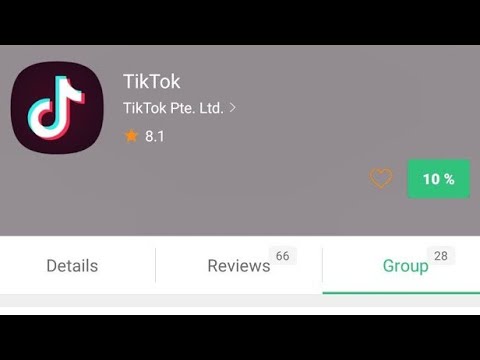The image showcases a screenshot featuring a rectangular screen with distinct horizontal black lines at the top and bottom, serving as a header and a footer. Just below the top black header is a solid gray rectangle. On the upper left corner within this gray rectangle is the TikTok logo, which consists of the colors white, red, and blue, set against a black square background. To the right of the logo, white text reads "TikTok, TikTok PTE. Limited," followed by a right-pointing arrow.

Directly beneath this text, there is a yellow star, next to which the number "8.1" is displayed. In the lower right corner of this gray rectangle is a green box containing white text that reads "10%", accompanied by a heart symbol to its left.

Below this section is a white banner with text that reads "Details" and "Reviews" from left to right. On the upper right corner of the "Reviews" section is the number "66." Additionally, the word "Group," written in green text and underlined, is also present, with the number "28" positioned in the upper right corner of the word "Group."